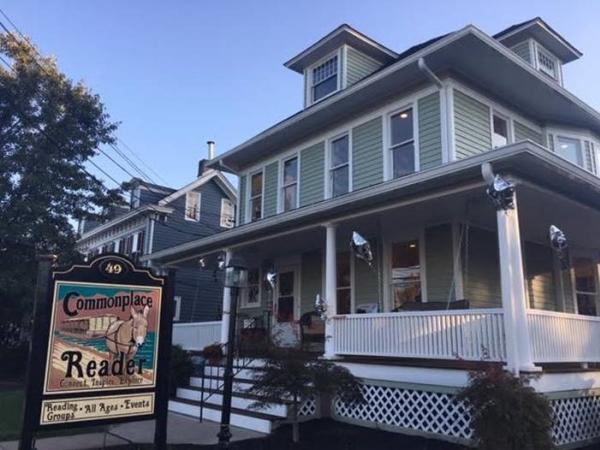The image depicts a clear, bright daytime view of a semi-colonial style house, primarily painted in lime green with white siding and window borders. The house features three floors including a possible attic space, indicated by single windows on both the topmost level and the other side of the house. The main façade includes four rectangular windows on both the lower and upper levels. Leading up to the front porch, there are white stairs flanked by a white railing. 

In the lower left corner of the image, a ground-mounted sign reads "Commonplace Reader" with an illustration of a horse, possibly a donkey, in harness between the words. Below the main text, the sign further advertises "Reading Groups, All Ages, Events," though some details are somewhat ambiguous. The number "49" is also visible on the sign. The house is elevated, with a white picket fence-like structure at the base, and surrounded by greenery including small trees and a large tree with green leaves to the left. 

To the left of the green house, another similarly sized dark gray house is visible, indicating a residential town setting. The image is well-lit by natural light, with a clear blue sky above and no people or vehicles in sight.